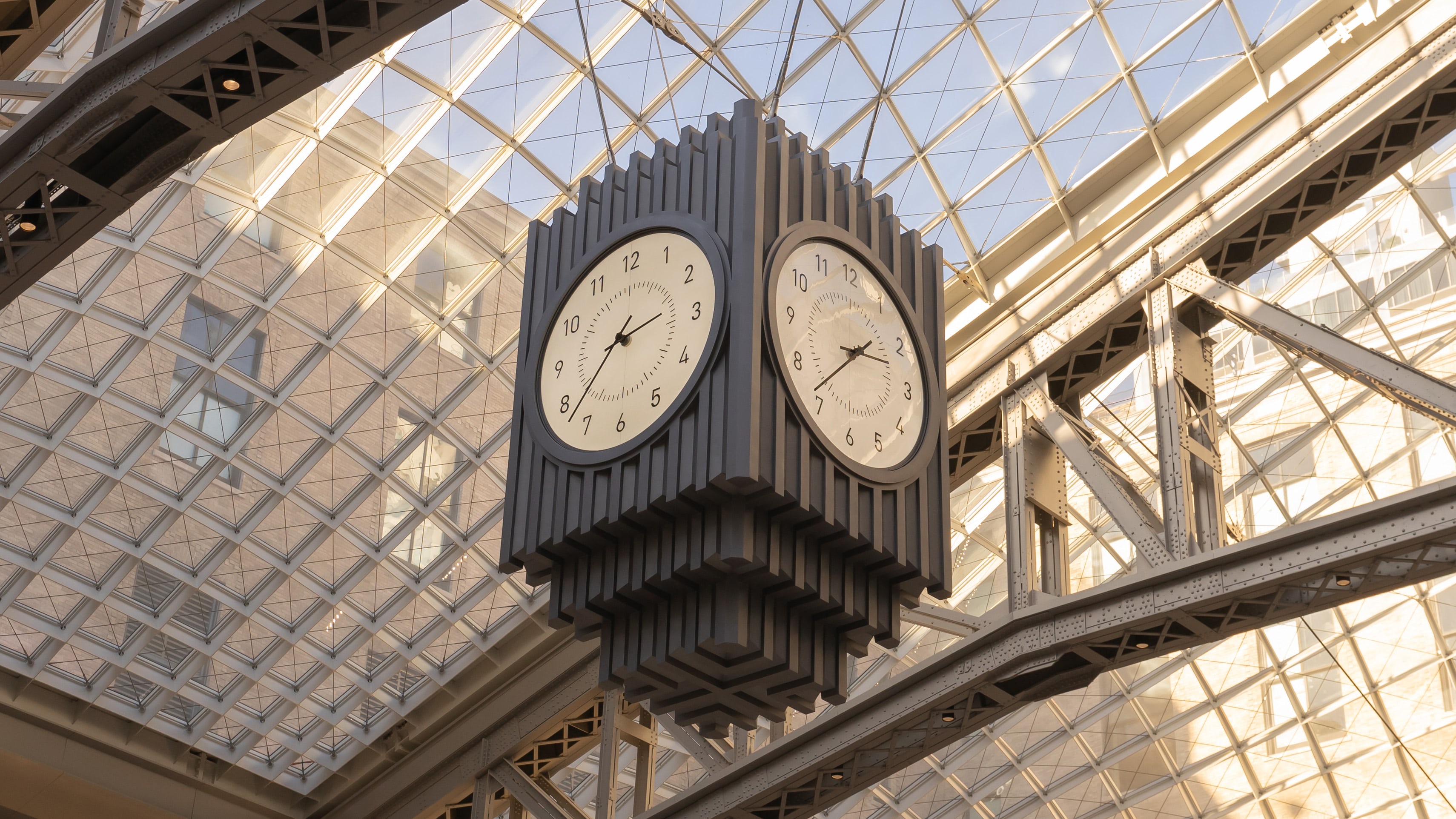In this close-up photograph, a large wooden clock is prominently suspended from the ceiling in the center of a spacious lobby or train station. The architectural marvel of the building features a roof composed of a metal and glass structure, giving it a transparent, waffle-like texture that allows a clear view of the sky. This pattern extends vertically down the sides of the edifice, supported by visible metal trusses and beams. The clock, which has a square design, displays the time 2:38 PM on each of its four faces. The building's ceiling is essentially a massive skylight made up of numerous small square glass windows that bathe the interior in natural sunlight. Through the glass, you can see the outlines of adjacent buildings, including a tall brick building and another structure to the right, suggesting the venue is located in a bustling downtown area. The detailed craftsmanship and strategic placement of the clock make it a central visual and functional focal point within this grand, light-filled space.